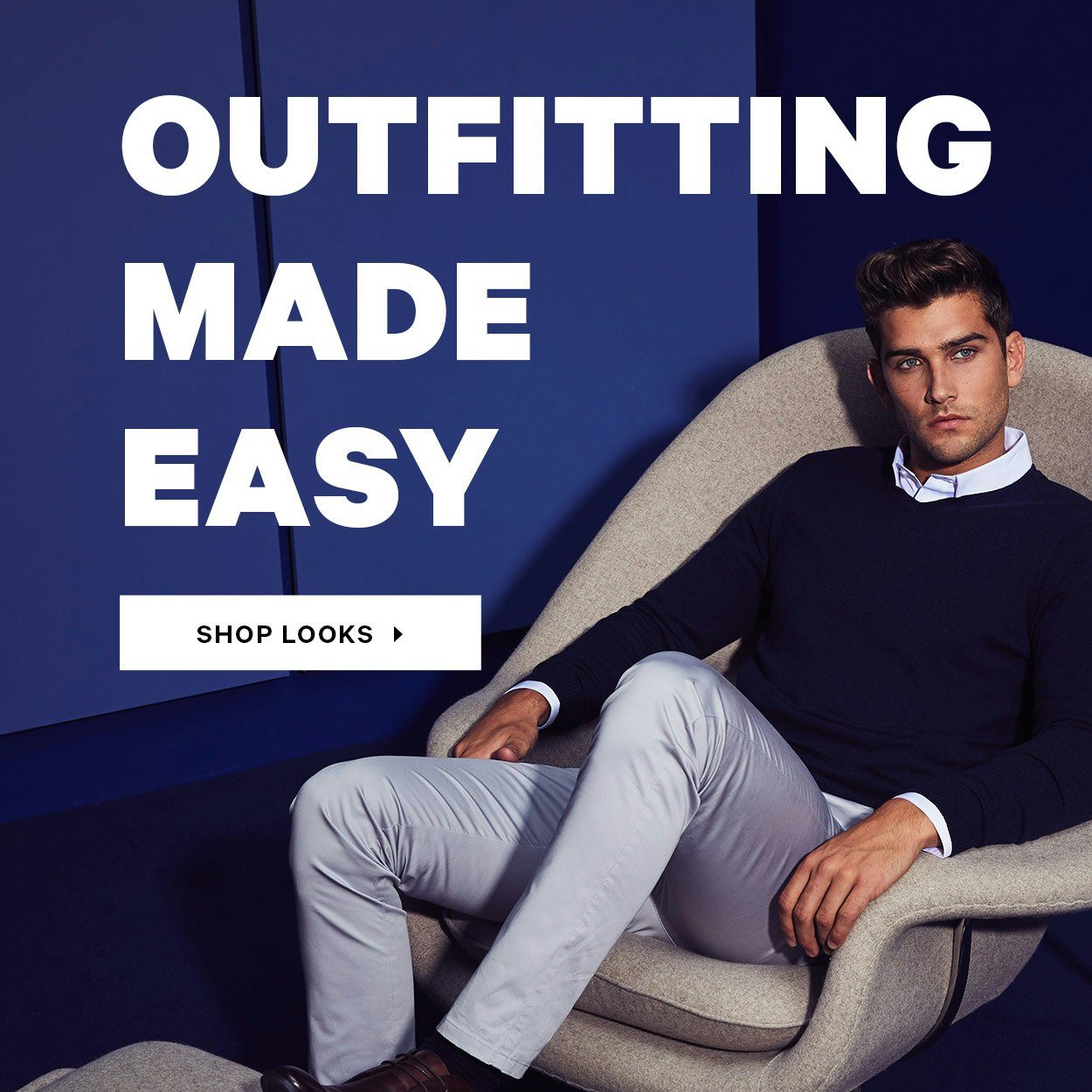In this advertisement image for a clothing company, a young brunette gentleman, approximately 25 years old, is the focus. Seated in a modern beige chair against a blue wall background, he radiates a blend of casual and professional style. He wears a crisp white collared shirt under a navy blue v-neck lightweight sweater, with the white sleeve cuffs emerging at the wrists. His outfit is completed with tailored light gray silky tapered pants and brown leather shoes. One foot is propped up on a matching ottoman, adding a relaxed demeanor to his poised appearance. The left side of the image features bold white text that reads, "Outfitting Made Easy," each word on its own line. Below is a white horizontal text box with black text inside that reads, "Shop Looks," accompanied by a rightward pointing arrow. The composition suggests a modern, sophisticated look, making it suitable for a banner ad or a company website. The photograph, rendered in a square format, showcases different shades of blue, white, gray, tan, brown, and silver.